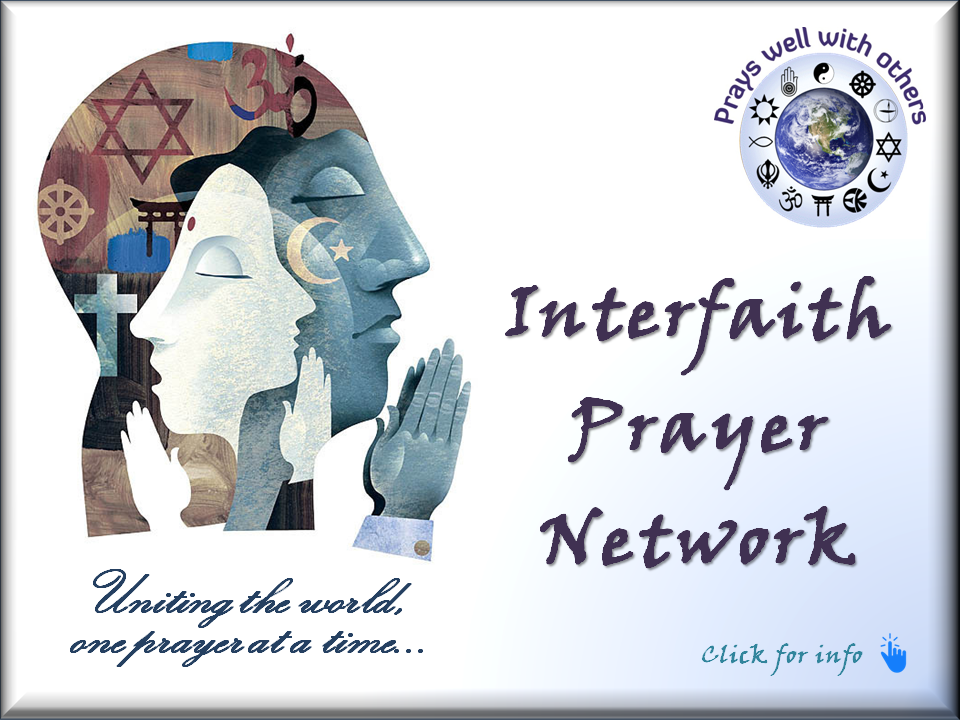The image appears to be a digital poster resembling a framed signboard, with a gray outer frame and a white and gray gradient background. On the left side, there is an intricate design featuring overlapping silhouettes of three faces within one another, all pointing to the right with clasped hands in a prayer gesture in front of them. These faces, presenting elements of both male and female features, and the hands, adorned with a range of symbols representing various religions including Judaism, Christianity, Islam, and Hinduism.

Near the bottom of this imagery, there is a cursive tagline that reads, "Uniting the world, one prayer at a time...". To the right side of the poster, the header "Interfaith Prayer Network" is prominently displayed at the center. Below this, in the bottom right corner, is a clickable area with an image of a blue hand and the instruction "Click for more info."

In the top right corner, a circular logo features the Earth at its center, encircled by symbols from numerous religions like Hinduism, Islam, Christianity, and Sikhism, accompanied by the phrase "Pray well with others."